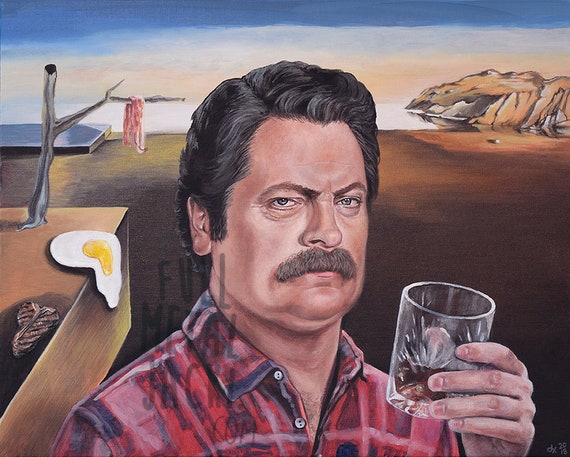This painting is a humorous and abstract portrayal of Nick Offerman as his iconic character Ron Swanson. Dominating the foreground is a detailed depiction of Ron Swanson, characterized by his thick, bushy mustache and neatly combed, wavy hair. He wears a red plaid flannel shirt and is holding a clear glass of what seems to be scotch whiskey near his face, which sports a stern, piercing gaze directed outward.

In true Salvador Dali-like fashion, the painting features a surreal and abstract background. A dead tree branch emerges from a table to Ron's left, draped with an unusual pink piece of fabric, reminiscent of bacon. Also on the table is a Dali-esque fried egg in the midst of sliding off the edge. The landscape in the background includes a desert-like setting with a blue-gray sky streaked with clouds, clear water, and a distant cliffside. To the far right, there's a more discernible brown mountain, adding to the fantastical scene.

Additional details include what might be a signature at the bottom of the painting, possibly reading "DK 2018," and faint text across part of Ron's image that appears to advertise "FullmetalJackie.com," suggesting a connection to the artist’s website. The overall composition blends the arresting presence of Ron Swanson with whimsical and dreamlike elements, creating a striking and amusing piece of art.